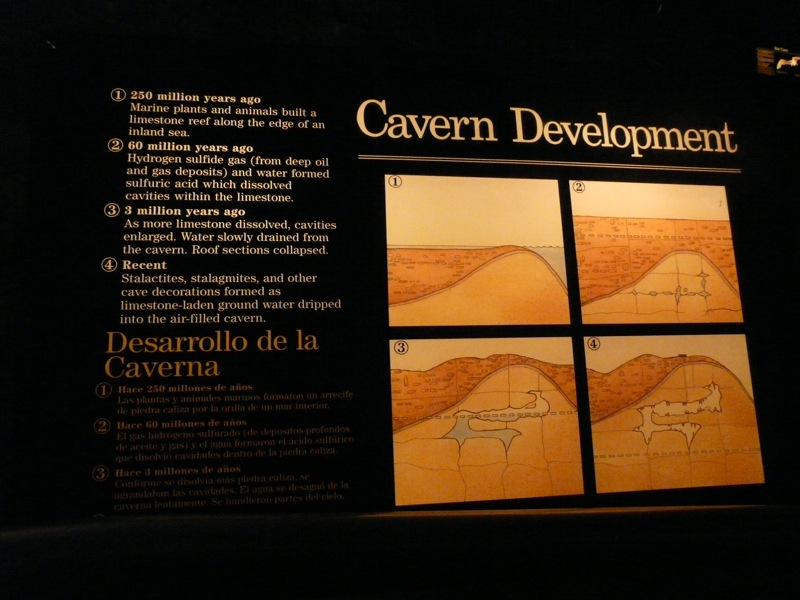This image is of an informational display for cavern development, set against a black background. The lit display contrasts with the dark surroundings, drawing attention to its content. On the left side, the display features four paragraphs of text labeled 1, 2, 3, and 4. These sections describe a chronological sequence: 

1. "250 million years ago, marine plants and animals built a limestone reef around the edge of an inland sea."
2. "60 million years ago, hydrogen sulfide gas from deep oil and gas deposits combined with water to form sulfuric acid, which dissolved cavities within the limestone."
3. "3 million years ago, as more limestone dissolved and cavities enlarged, water slowly drained from the cavern, causing roof sections to collapse."
4. "More recently, stalactites, stalagmites, and other cave formations developed as limestone-laden groundwater dripped into the air-filled cavern."

The same information appears beneath this, but written in Spanish under a heading labeled "Di Sarolo della Caverna".

To the right of this text, the display header "Cavern Development" stands out in bright yellow. Below this header are four quadrants showing cross-sectional images of cavern development over time: 

- The top left image shows a lot of dark color at the top with light at the bottom.
- The bottom left image features less dark at the top and more light beneath.
- The top right image displays a large dark area on the top with a smaller light portion below.
- The bottom right image has minimal dark area on top with a large light area below.

There is also a symbol or icon above and to the right of the display that isn't clearly visible. The overall presentation is framed by black space, accentuating the lit-up detail of the displayed information.